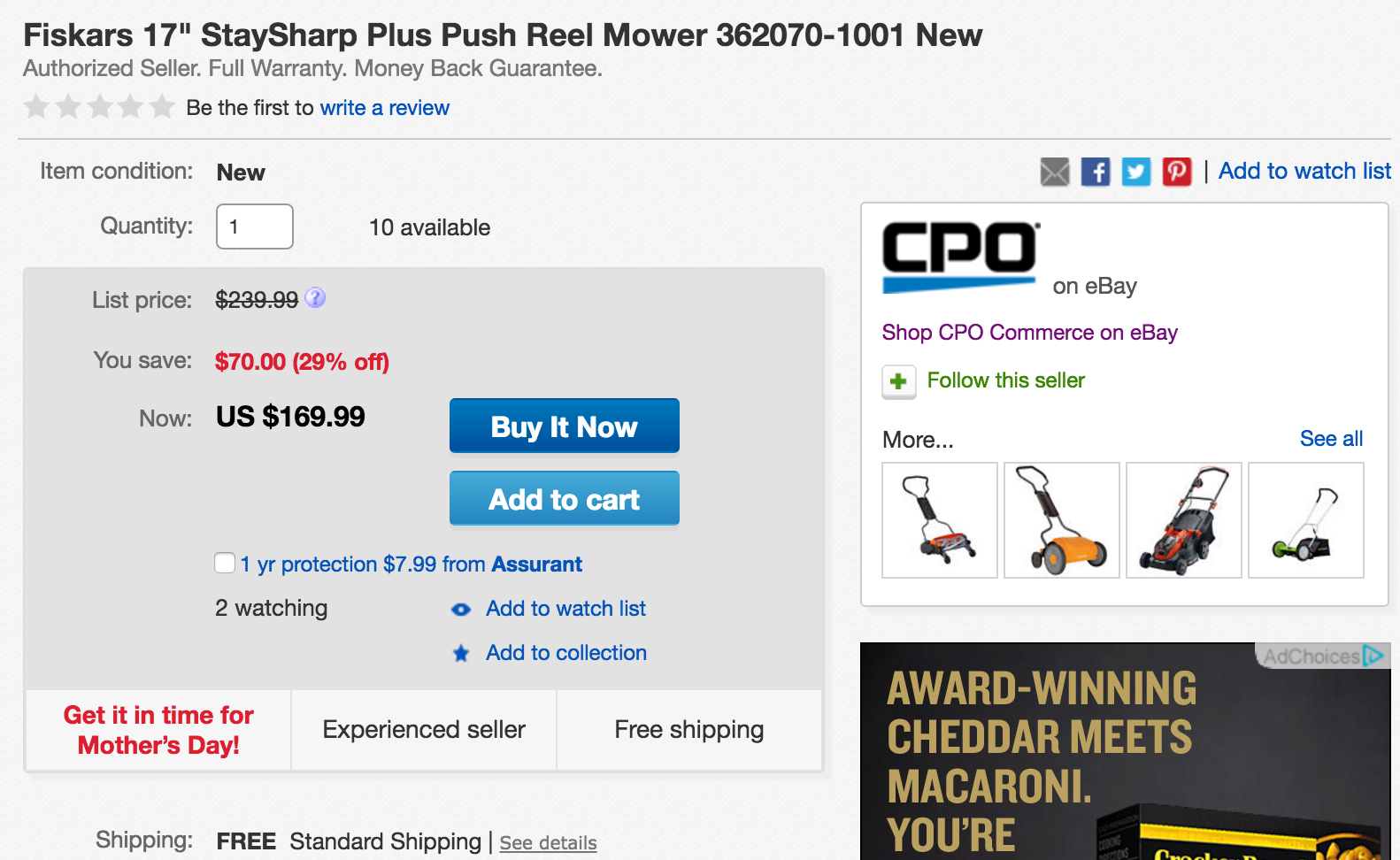Screenshot Description:

The image captures an e-commerce listing for a Fiskars 17-inch StaySharp Plus Push Reel Mower (model 3620 70-101). At the top of the listing, the product name and model are prominently displayed. Below, it indicates that the item is sold by an authorized seller, featuring a full warranty and a money-back guarantee. There are five empty stars shown for the product rating, suggesting there are no reviews yet.

Additional product details include:
- Item Condition: New
- Quantity Available: 1 to 10
- Original List Price: $239.99
- Current Price: $169.99 (a savings of $70 or 29% off)

On the right side of the screen, there are two call-to-action buttons: a dark blue "Buy It Now" button and a light blue "Add to Cart" button. Beneath these, it offers a one-year protection plan from Assurant for $7.99.

Two potential customer actions are noted as well: adding the item to a watch list or a collection. 

Lastly, a note indicates that this item is being promoted in time for Mother's Day.